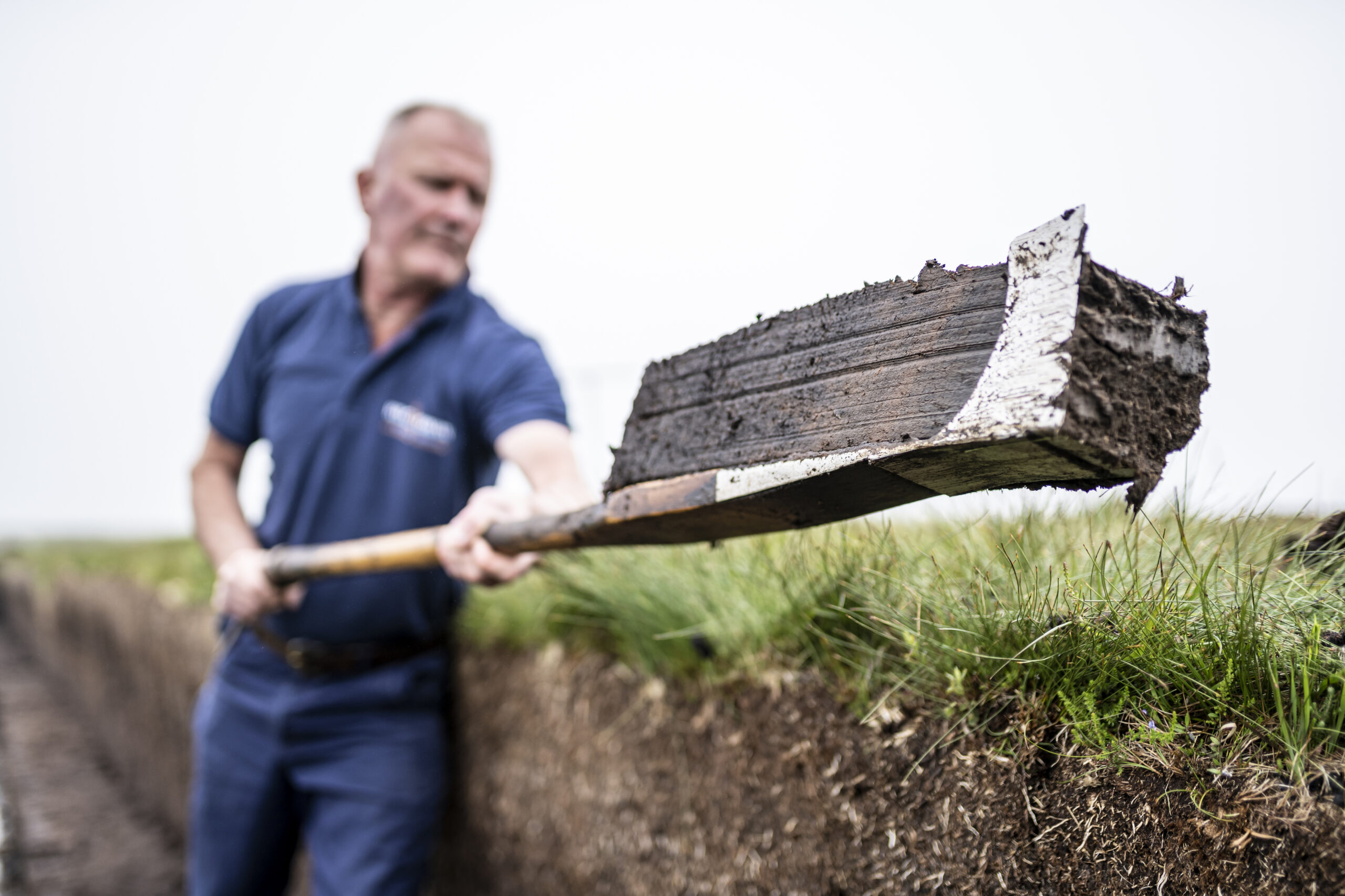In this detailed outdoor scene, an older white man with short, gray hair and a reddish complexion is depicted mid-dig, using a specialized rectangular-ended tool. He is centered to the left side of the frame, dressed in a dark blue t-shirt, blue jeans, and a brown belt. Holding the tool with both hands, his left hand is extended while his right remains near his body. The tool is lifting a perfectly cut rectangular piece of black dirt, creating a distinct and in-focus focal point towards the middle-right of the image. Behind him, a neatly dug trench is visible, lined by a wall of dark soil with grass growing on the upper edge, angled diagonally, adding depth to the scene. The background gradually blurs, emphasizing the man's action and the tool with the dirt wedge as the primary subject.